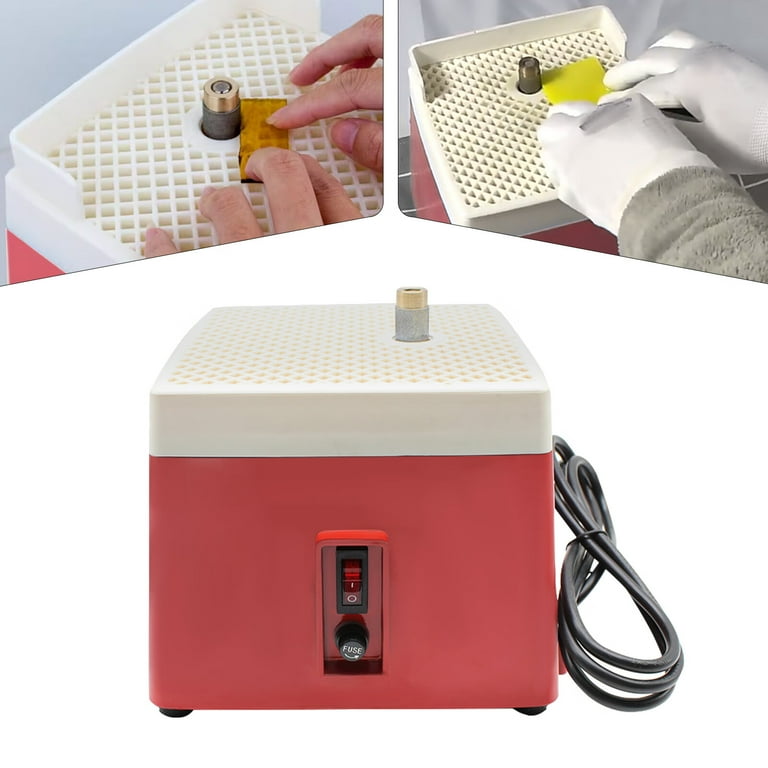The image comprises three professionally composed photographs arranged with a white background, depicting an electronic device with a red base and a white top. Central to the images, at the bottom, the device features a dark red power switch labeled with an "I" and "O" indicating on and off positions, and a black knob labeled "Fuse" with a white arrow pointing to the right. A black cable extends from the right side of the device. The top surface of the device has multiple recesses, including a prominent circular one housing a metal object or cylindrical component.

In the top left photograph, a person is placing a clear amber-colored plate against the metal object protruding from the circular recess. Meanwhile, the top right photograph shows the same person, this time wearing white gloves, positioning a yellow plate against either the same or a different metal object in the same recess. The overall composition and high-quality appearance of the image suggest it is intended for an advertisement, yet the specific function of the device remains ambiguous.